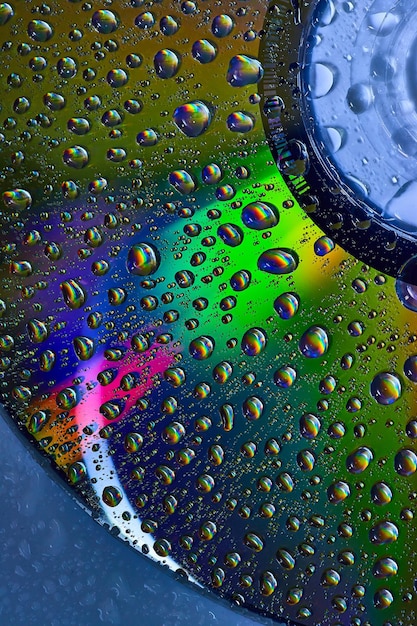This color photograph depicts a highly detailed, close-up view of the underside of a compact disc (CD) sprinkled with water droplets. The image primarily focuses on these water droplets, each of which contains a tiny reflection and refraction of rainbow colors due to the light interacting with the CD's surface. In the top right corner, a small part of the translucent central portion of the CD, along with a black strip adjacent to it, is visible. The CD surface in the background displays a vivid spectrum of colors, including gold, green, purple, and pink, emanating from the light's angle and the wet surface. The bottom left corner features part of a blue surface also dotted with water droplets. The photograph lacks any visible writing, people, animals, or structures, keeping the intricate details of the water droplets and the CD's colorful reflections as the focal points of this mesmerizing image.